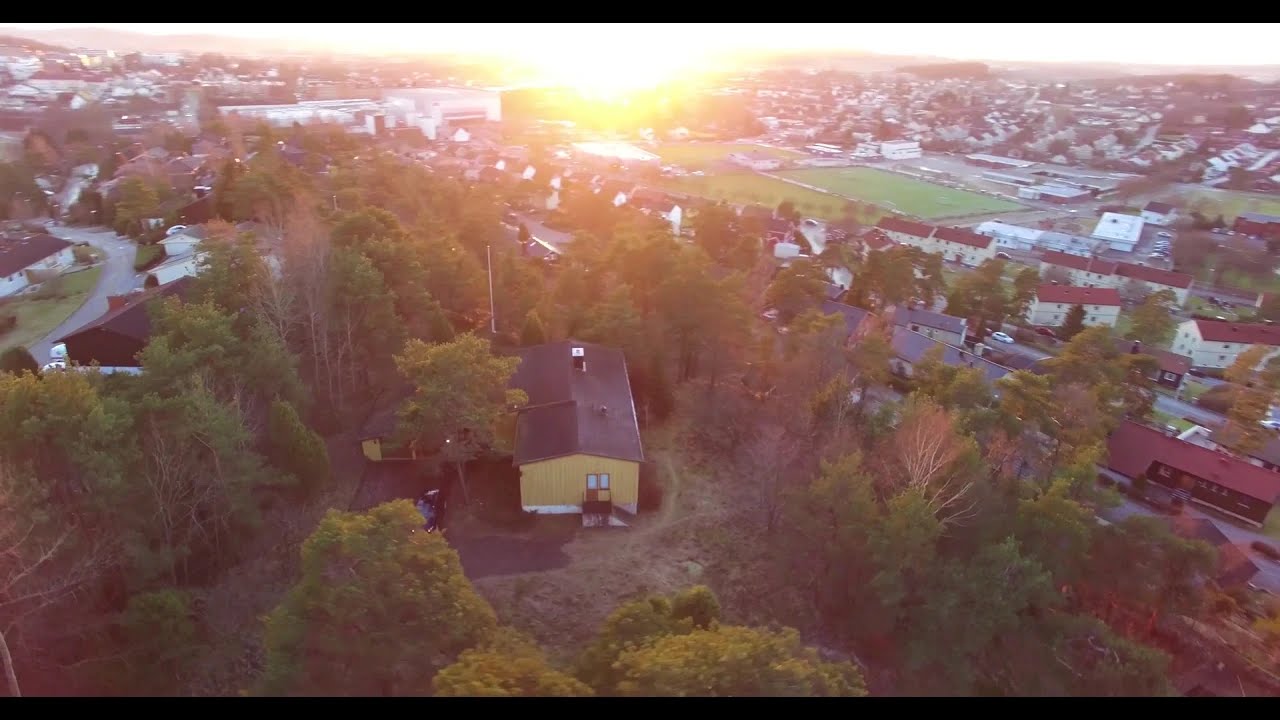The photograph captures a breathtaking sunset view of a suburban town from a slightly elevated vantage. At the center of the image sits a light yellow house with vertical siding, accented with white trim and crowned by a black, sloped roof. The house, featuring a sizable two-car garage on the left with a car parked in the driveway, is nestled amidst tall, dense trees, giving it a somewhat secluded feel.

To the left of this house, a street winds past a few houses, blending seamlessly into the scene. The right side is characterized by a suburb of densely packed buildings with a mix of red and gray roofs. In the foreground, the houses give way to expansive green fields, punctuated by a football field and larger commercial buildings such as warehouses or retail parks further in the background.

The sun, positioned at the top center of the photograph, glows intensely, casting a radiant light that gradually softens the scene and extends into the distant horizon, where rows of suburban homes and additional greenery paint a picturesque backdrop.